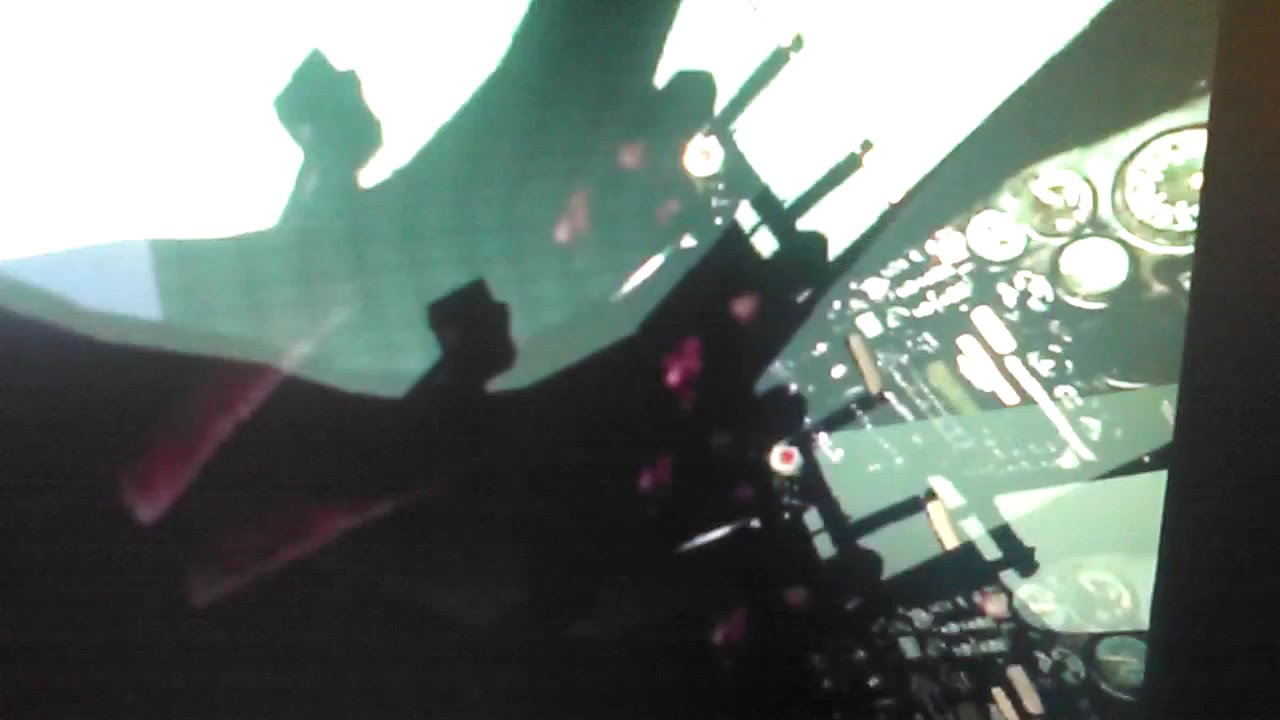This image is a low-quality, rectangular photo, approximately six inches wide by three inches tall, depicting a cluttered scene that strongly suggests the interior of an aircraft, possibly a small plane cockpit. The upper left-hand corner of the photo is obscured by a significant glare, likely due to direct sunlight, which washes out part of the image and adds to the overall blurriness. A beam of white light penetrates from this corner, casting a curved shadow and contributing to the reflections that muddle the perception of the scene.

In the foreground, tilted on its side, there appears to be a console panel adorned with myriad gauges, dials, and knobs. The panel is situated more prominently on the right-hand side, featuring a mix of black, white, light blue, green, red, pink, yellow, and tan colors, which may correspond to various indicators and alerts typical within a cockpit. Additionally, the image shows reflections, potentially of individuals or nearby buildings, making it harder to discern the specific layout and details.

To the left, an area predominantly red and another predominantly green are visible, along with rods that evoke the impression of upturned chair legs. This left section also contains something that might resemble a human fist being raised, though the exact nature is unclear due to the photo's poor quality. Beyond the cockpit, a reflection of what appears to be the sky, in white and blue hues, can be observed, reinforcing the notion of an aerial setting and enhancing the sense of looking through a transparent material, like glass, into the vast expanse outside.